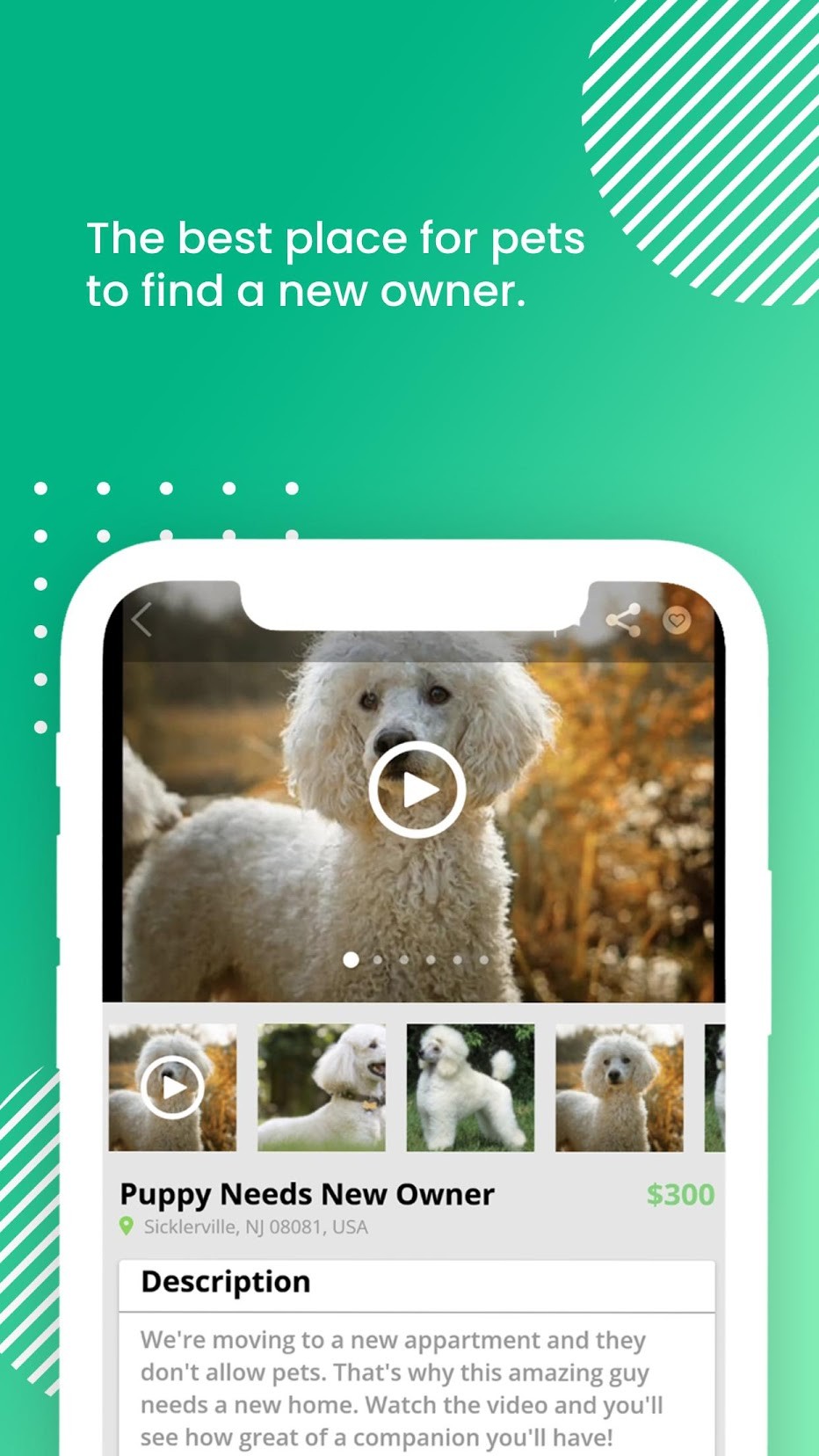On a vibrant green background, a video displays detailed information concerning a dog in need of a new owner. At the top of the video, a white text banner reads, "The best place for pets to find a new owner." An image of a dog, symbolizing the video content, is placed next to this text.

In the middle section, a caption specifies that a puppy, valued at $300, is seeking a new owner. The location "Sicklerville, New Jersey 08081, USA" is noted beneath this information. The descriptive text below reads: "We're moving to a new apartment, and they don't allow pets. That's why this amazing guy needs a new home. Watch the video, and you'll see how great of a companion you'll have."

The featured dog is white and appears in a setting with a yellowish, possibly floral, background. Below the main image, four additional thumbnail-sized screens display various phases of the puppy's life, offering more visual snippets from the video.